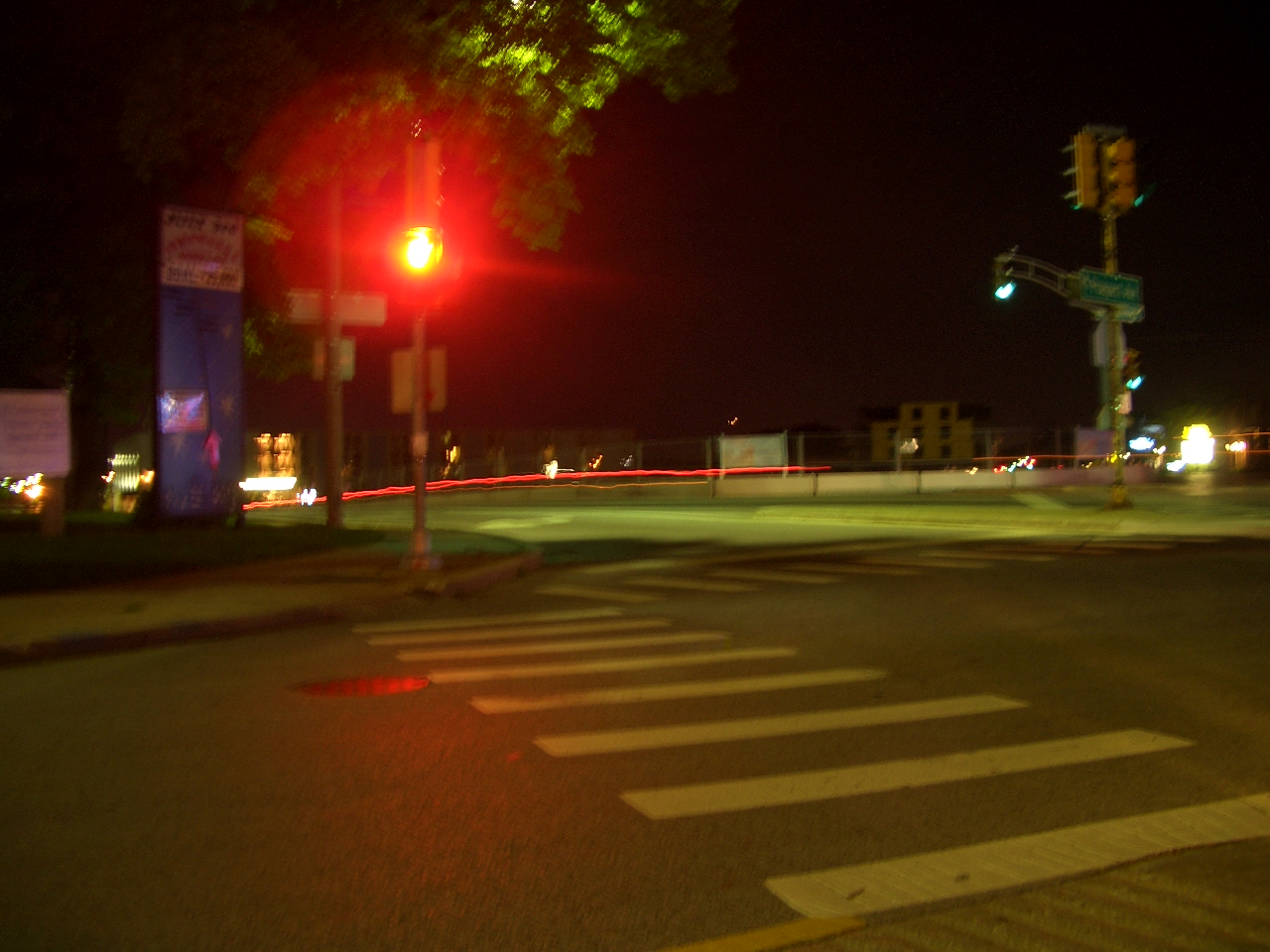The photograph captures a vivid nocturnal urban scene. It is taken on a street corner at night, with the central focus on a lone pole hosting a bright yellow streetlight, positioned slightly to the left. Surrounding the streetlight, a large, round red halo with red spikes radiates outward, casting an intense glow. Beneath this streetlight in the foreground, there is a crosswalk painted in yellow lines that stretches from the middle of the photograph towards the lower right edge, intersecting a diagonal part of the same walk heading towards the center edge. A sewer cap indicates a manhole near the end of this crosswalk.

Behind the crosswalk, there is a pavement and a blue building fragment, while a sign approximately 15 feet tall is situated to the left. The area features multiple taillight flares and additional small ground-level lights from buildings in the background. On the right side, there is a green-lawn area, likely adjacent to a tree with a slender but sturdy trunk and an abundance of green leaves. Midway up the right-hand side, what appears to be a green crane is illuminated halfway up its structure, with scattered lights around it. Towards the back of this lawn area lies a band of red, possibly a neon light or barrier.

Above the halo of the streetlight, one can observe some tree tops against the backdrop of a pitch-black sky, adding a natural element to the urban setting. Additionally, there are two more traffic lights and another streetlight visible in this intricate, meticulously illuminated night time street scene.